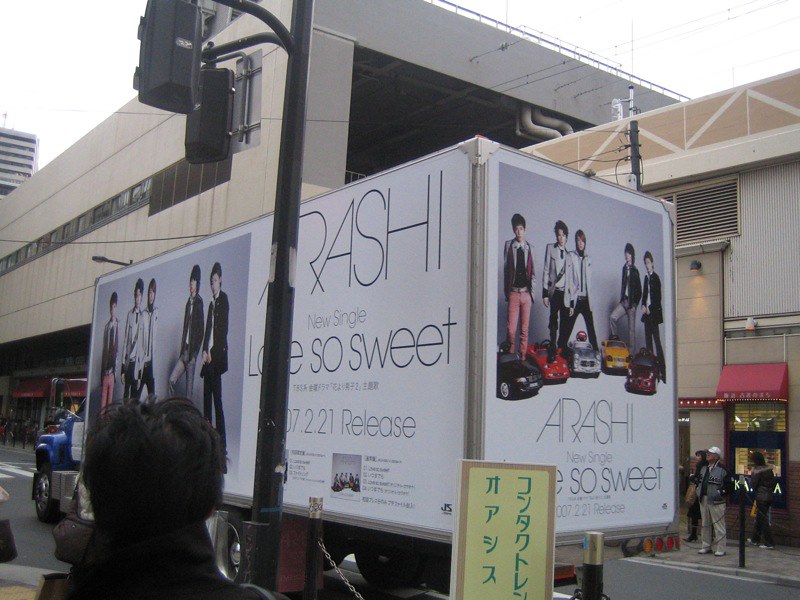The scene captures a bustling urban street in a Japanese city, where a semi-trailer truck, predominantly white with a deep blue cab, is parked alongside the road. The truck features an advertisement promoting the band Arashi and their new single "Love So Sweet," released on July 21, 2021. The side and back panels of the trailer display an image of five well-dressed band members in suits, with "Arashi" and "Love So Sweet" prominently written. Additionally, the back panel beneath the band members shows cars in black, red, silver, yellow, and burgundy. The scene includes several onlookers gathered near the truck, possibly in front of a shop, creating a lively atmosphere. In the background, there are notable structures, including a large white building with horizontal windows and a shopping center-style building, along with traffic lights and other elements typical of a busy cityscape.